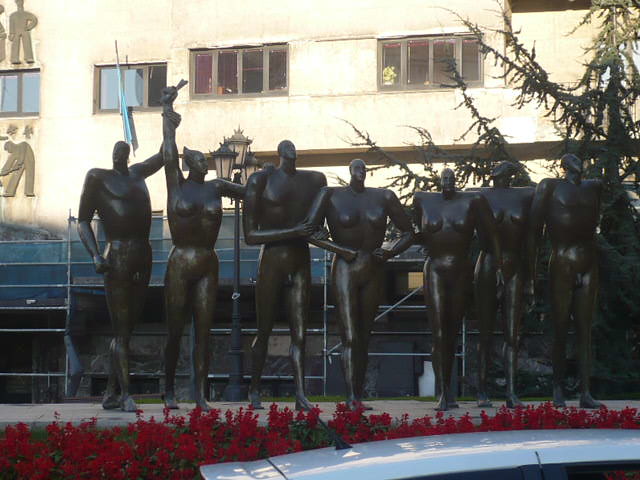The photograph captures a striking outdoor scene with seven elongated, dark bronze statues positioned horizontally from left to right. These statues alternate between male and female forms and are depicted with exaggeratedly long legs, barrel-like chests, and proportionately small heads. The first pair on the left, a male and female, are connected by their elevated arms in a gesture of triumph. The other figures show varied poses, some with hands on their hips and others with arms crossed over their chests. They are arranged on a cement pedestal adorned with a border of vibrant red flowers. Behind the statues stands an older tan building, likely stucco, featuring high, dark windows and architectural figurines on its walls. A parked car can be seen at the base of the pedestal, adding a touch of everyday life to this evocative scene.